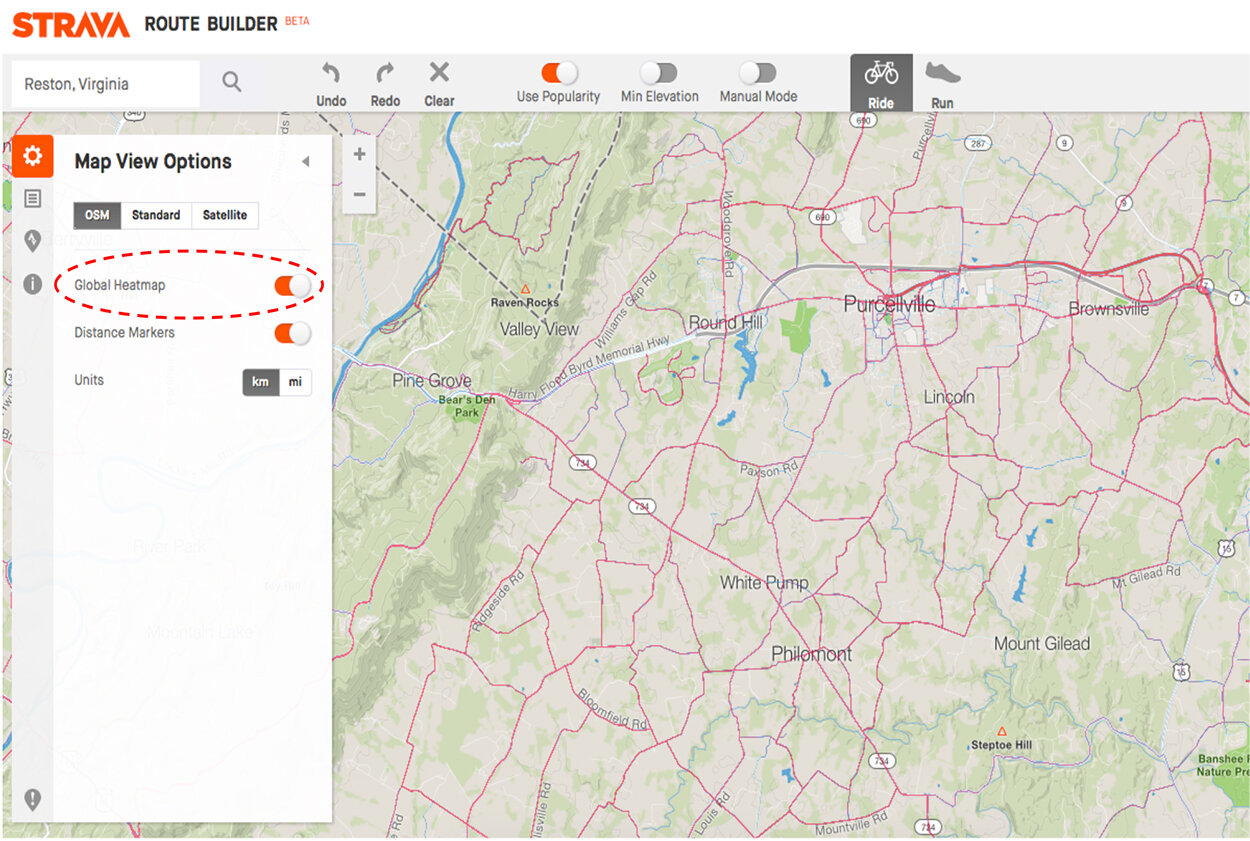A screenshot of a website related to maps is presented, identified at the top with the orange text "Strava" followed by black text "Route Builder" and an orange "Beta" label. Below the header, a white search box displays "Reston, Virginia" accompanied by a gray magnifying glass icon. Adjacent to it, there are gray "Undo", "Redo", and "Clear" buttons, each labeled accordingly. 

Below these controls, a row of circular buttons is shown: an orange and white button labeled "Use Popularity," and two gray and white buttons labeled "Min Elevation" and "Manual Mode." To the side, there are icons representing different activity modes: a bicycle icon labeled "Ride" within a gray box, and a shoe icon labeled "Run."

On the left side of the screen, a white sidebar contains several icons: an orange and white cogwheel, a gray paper icon, a gray location pin icon, and a gray circle with an "i," collectively labeled as "Map View Options" in black text. Below this, there are three map style options: "OSM" in gray and white, and "Standard" and "Satellite" in black and white boxes. A highlighted option, "Global Heatmap," is circled in orange. Another option, "Distance Markers," is presented in a white and orange circle. Further down, there is an option to toggle units between kilometers (KM) and miles (MI), with KM currently selected.

The map itself features a mix of white and green terrain with numerous purple routes. Key locations indicated on the map include Lincoln, Brownsville, White Pump Hill, Mount Gilead, Raven Rocks, Pine Grove, and Valley View, along with various labeled roads and blue water bodies visible on the map.